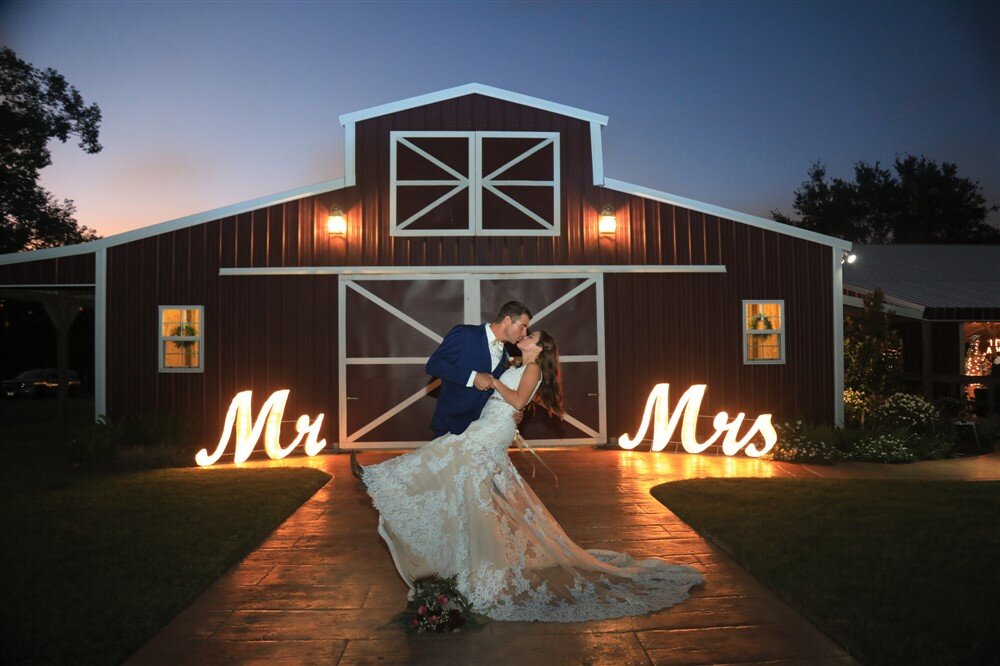In this captivating, high-quality wedding photo taken during twilight, a newly married couple shares a loving kiss in front of a dark red barn. The barn, serving as the wedding venue, is warmly lit by glowing yellow lights and lanterns on either side. The illuminated cursive signs reading "Mr." and "Mrs." frame the couple, adding to the romantic ambiance. The bride, adorned in a lacy white wedding gown with a long trail, has her bouquet tossed to the ground as she kicks up one cowboy-boot-clad foot while leaning back into her husband's arms. The groom is elegantly dressed in a tuxedo, creating a timeless and heartwarming scene of newlywed bliss.